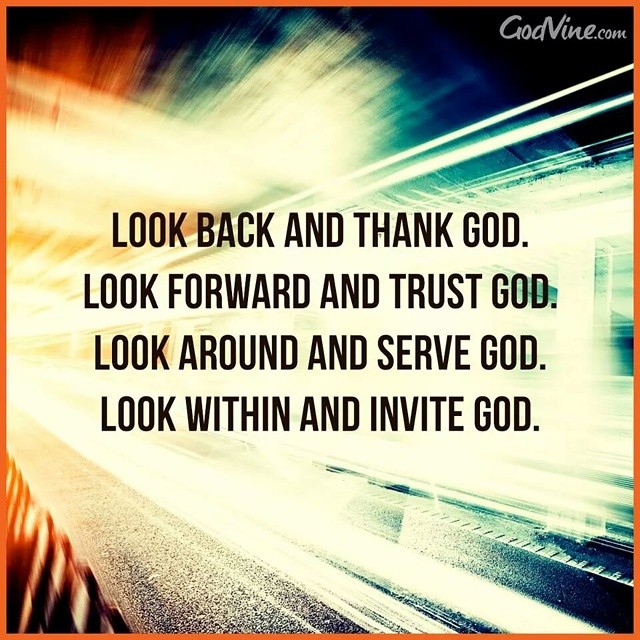This image features an inspirational poster with a powerful religious message. The poster is square with a thin bronze border, and the focal point is a quote in large, black, uppercase font that is centered both horizontally and vertically. The quote reads: "Look back and thank God. Look forward and trust God. Look around and serve God. Look within and invite God." The background of the image showcases a radiant shaft of light, resembling beams of light in a subway or railroad station, adding a dynamic effect. The border includes various shades of orange and blue, contributing to the overall vibrant appearance of the poster. In the upper right corner, there is a mention of "Godvine.com," indicating a source for more inspirational content. This beautifully designed image serves as a reminder to reflect on one's faith and gratitude.